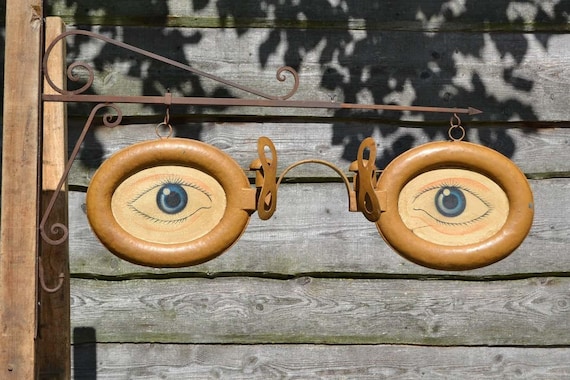An old-fashioned sign for eyeglasses is mounted on the left side of a weathered wooden building with horizontal planks. The sign comprises a rusted metal pole with intricate filigree work and an arrow pointing to the right. Suspended from the pole is a life-sized pair of ornate, oval eyeglasses. The glasses are depicted with tan frames and feature blue eyes painted within each lens, complete with short eyelashes and matching highlights in the pupils. The metal frame includes an arch with two pads mimicking the nose pads of traditional glasses. A shadow of leaves casts down over the scene, emphasizing the vintage charm of this eyeglass sign, likely indicative of an old optometry office.